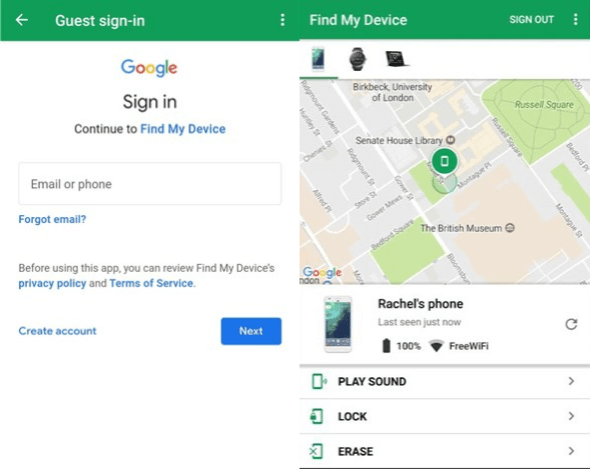Here is a cleaned-up and detailed caption for the image:

---

The image is a screenshot from a website featuring Google's "Find My Device" service. At the top of the page, there is a thick green bar stretching across the width. On the left side of this bar, a white arrow points left, followed by the text "Guest sign-in" in white, with a dash separating "sign" and "in." Centrally aligned within the bar are three vertically stacked white dots. To the right, it reads "Find My Device" in white text, followed by "Sign out." Another set of vertical dots is positioned at the far right of the green bar.

Beneath the green bar, in the top center, "Google" is displayed with multi-colored letters: G in blue, O in red, O in yellow, G in blue, L in green, and E in red. Directly below, the black text reads "Sign in," followed by "Continue to" and the blue text "Find My Device." Below this, there is a white input bar with black text inside that reads "Email or phone."

Further down, "Forgot email?" is clickable in blue on the left, followed by the black text: "Before using this app, you can review Find My Device's Privacy Policy and Terms of Service," where "Privacy Policy" and "Terms of Service" are in blue. Below this, "Create account" is in blue on the left while a blue "Next" button with white text is on the right.

On the right-hand side of the page, there are images of a black phone, a black watch, and a black laptop. The phone is highlighted with a green underline. Below these images is a map displaying locations including "Birkbeck University of London," "Senate House Library," and "The British Museum."

Further down, an image of a white phone labeled "Rachel's phone" indicates it was "Last seen just now." A black battery icon showing 100% is followed by a Wi-Fi signal icon with the text "Free Wi-Fi" in black. Below this section, a green phone icon next to "Play sound" is followed by another green phone icon with a green padlock and the text "Lock." Finally, a green phone icon with a green X next to it is followed by the word "Erase."

---

This caption provides a comprehensive description of all visual and textual elements in the image.